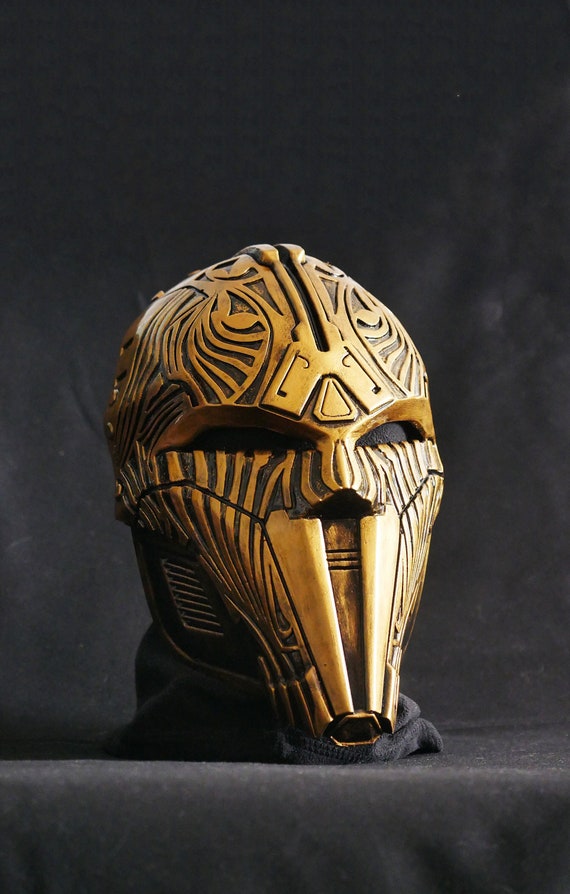The image is a full-color, vertically rectangular photograph of what appears to be a meticulously staged display of an ancient artifact or museum piece. Set against a backdrop of black cloth that drapes both the background and the surface it's placed on, this display prominently features a striking gold helmet with intricate black line motifs resembling tiger stripes. The overall design of the helmet is symmetrical, with each side mirroring the other, and it sits atop what looks like a mannequin head. The eyes of the mannequin are covered with black material, adding to the sense of mystery. Notably, the mouth of the helmet is designed in such a way that it extends into two long, fang-like structures, reminiscent of a saber-toothed tiger. From the forehead up the middle of the head runs a black vertical line, further enhancing the helmet's elaborate design. The bottom of the mask is adorned with a black cloth, presumably to cover the neck, completing the artifact's dramatic and imposing appearance.